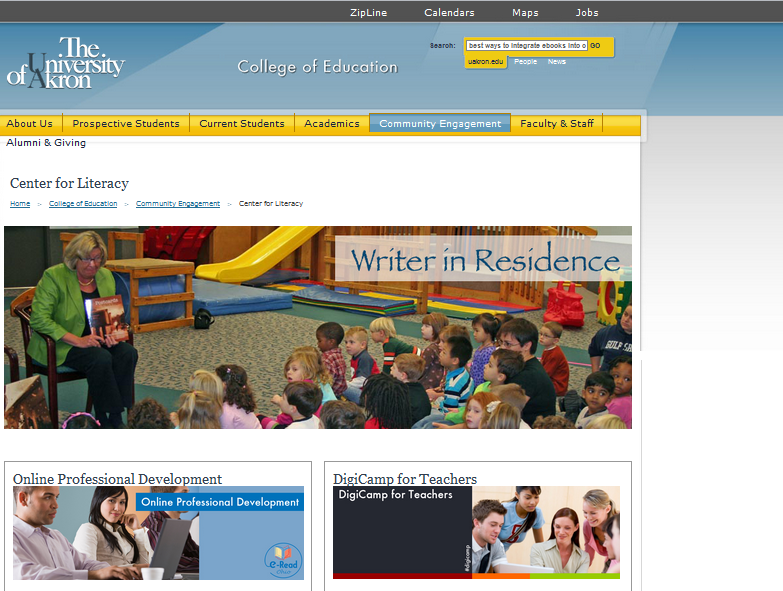The image is a screenshot of a desktop view of the University of Akron's College of Education website. The web address, browser, and operating system are not visible. The interface starts with a narrow gray bar at the top featuring options in white text: "Zip Line," "Calendars," "Maps," and "Jobs." Below this, there is a wider blue gradient bar which prominently displays "The University of Akron College of Education" in white uppercase letters.

A yellow-framed search bar with white text inside allows users to search the website, people, or news. Currently, the search term entered is "best ways to integrate e-books info."

Further down, there's a horizontal yellow menu bar with options for "About Us," "Prospective Students," "Current Students," "Academics," "Community Engagement," and "Faculty and Staff" in a bluish-black font. "Community Engagement" is highlighted in medium blue with white text, indicating the current section.

Beneath the menu bar are links reading "Alumni and Giving Center for Literacy" and "Home," reflecting navigation hierarchy: "College of Education > Community Engagement > Center for Literacy."

The main content showcases an older woman holding a book, engaging young children who appear to be in preschool or early elementary school. This section is labeled "Writer-in-Residence."

In the bottom-left corner, there is an image of people seated in what appears to be a classroom, accompanied by the text "Online Professional Development," which is repeated twice along with "e-Read."

On the right side of the page, another group of people is gathered around a laptop, labeled "Did You Camp for Teachers," which is also repeated twice.

This detailed view captures the essence of the College of Education's webpage at the University of Akron, focusing on its educational and community engagement offerings.